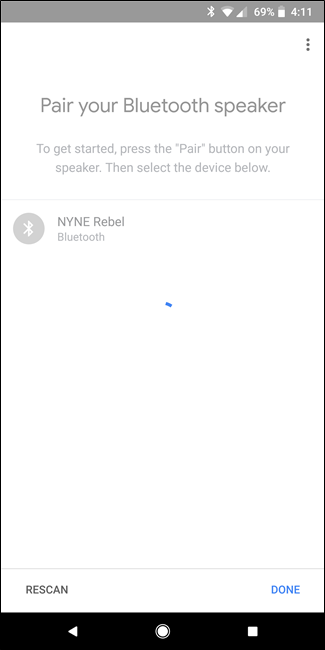The image displays a screenshot from a cell phone. At the top, there's a long, horizontal status bar in gray. On the right side of this bar, the battery life is shown at 69% in white text. Beside the battery icon, the time reads 4:11, also in white, indicating when the screenshot was taken. Directly beneath the time, there are three small white dots aligned vertically, each separated by a short distance.

Centered below this, in bold gray text, is the instruction "Pair Your Bluetooth Speaker." Further instructions in lighter gray text below read, "To get started, press the 'PAIR' button on your speaker. Then select the device below." 

Proceeding downwards, to the left, there's a gray circle with white lines inside of it. On the right, in all uppercase letters, is the label "NYNE REBEL". Directly beneath this label, the word "Bluetooth" is displayed.

At the bottom of the image, there are two options: "Re-scan" on the left, and "Done" on the right in blue text.